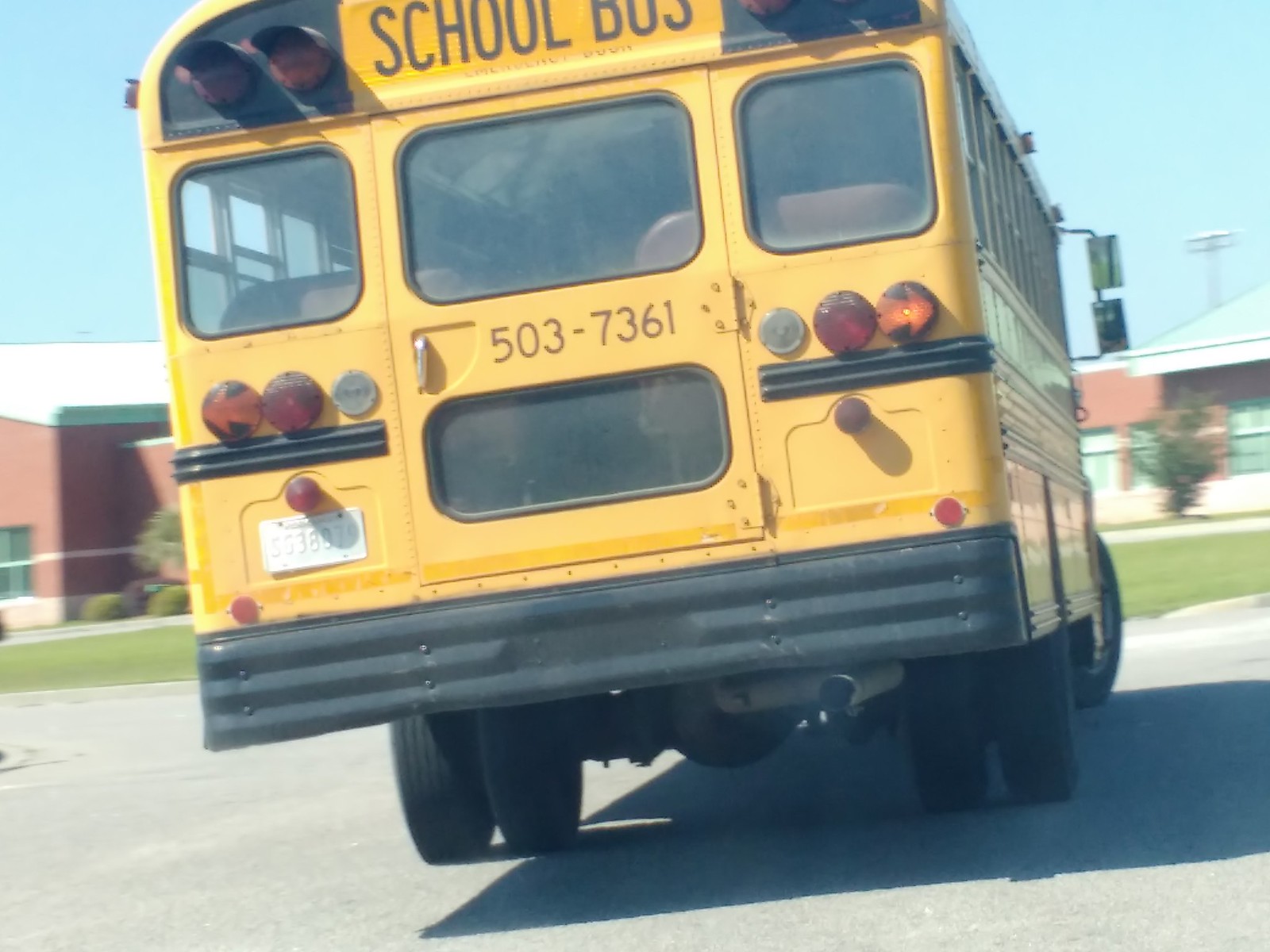In the image, a bright yellow school bus is prominently featured, captured from the back as it appears to be in motion, turning to the right. The bus is navigating a white asphalt street, adjacent to a verdant schoolyard. The rectangular brick school building, characterized by its green-accented windows, stands in the background under a very light blue sky. Stadium lights can be spotted far to the right of the scene.

The bus’s rear showcases several distinct details: three rounded corner windows evenly spaced across, including one that forms part of the central back door. Below the windows are three sets of red lights on either side, with an additional slightly smaller light beneath each set. The left light hovers above a white license plate embossed with black lettering. Centered on the door is the phone number 503-7361 in black text. The top back of the bus is marked with the words "SCHOOL BUS" in bold black paint. 

The bus's black bumper is substantial and sits towards the bottom left of the image, with an exhaust pipe visible, emitting a faint trail from the muffler. The rear wheels, four in total, are evident, with the right-side front wheel turned, reflecting the bus’s direction of movement. The overall scene emanates a sense of an everyday school routine, with the bus either arriving at or departing from the sizeable, serene school premises.